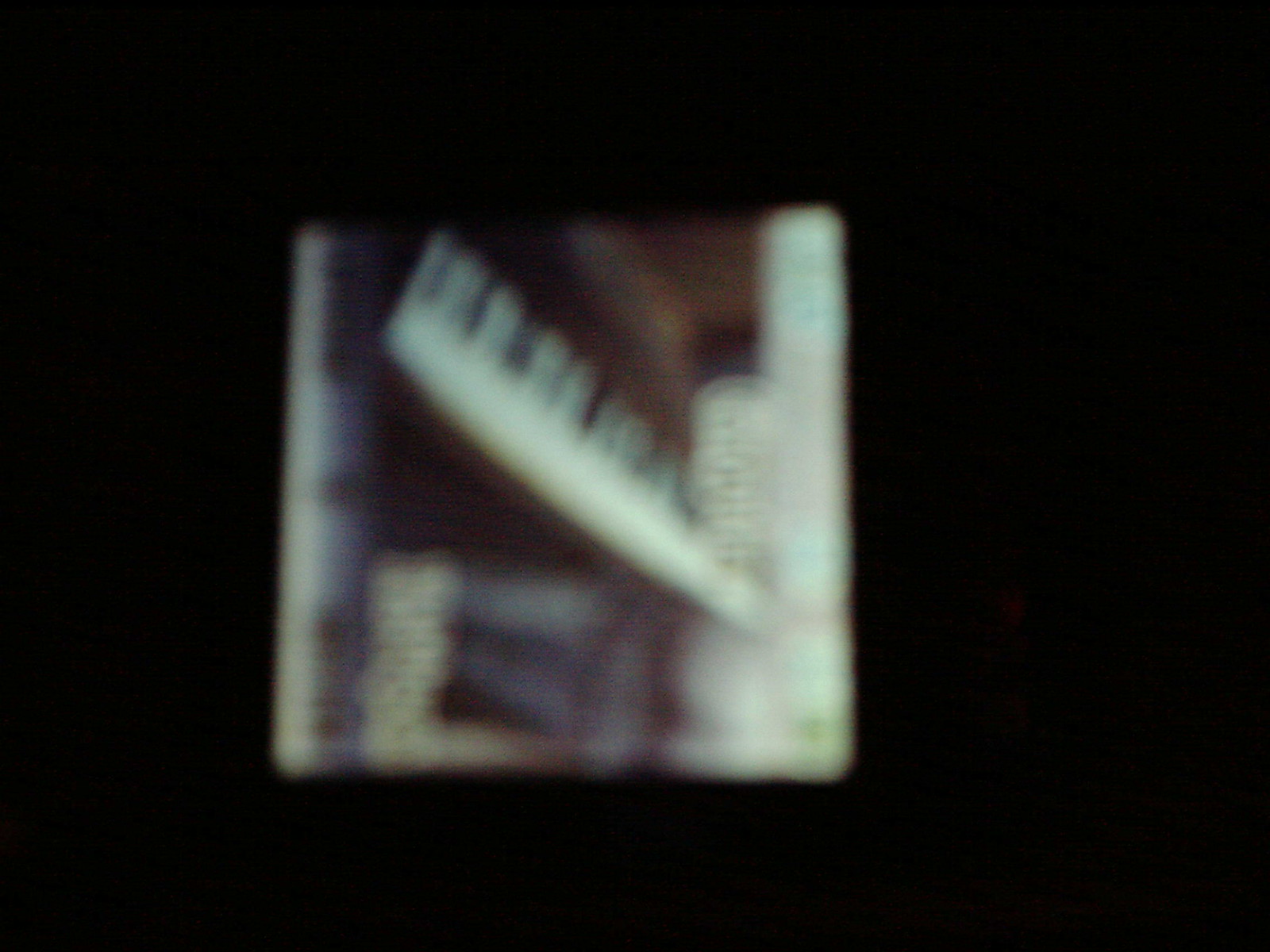In the very blurry and dark photograph, the backdrop is black, framing a predominantly square image positioned centrally. The image within the square appears to have a white border, with an indigo blue and black coloring blended, particularly at the edges. The center of this square is blurred but shows a mix of white and dark shades, potentially incorporating vertical light blue lines and obscure writing that isn’t legible due to the blur. There's also a faint suggestion of a brown tint in parts of the image, adding a slightly warmer tone amidst the overall dark and cool color palette. A mysterious long object, possibly resembling a white hairbrush with indistinct black and white bristles, can be faintly discerned in the middle. The left and right sides of the square are bordered by white lines, giving it a distinct, albeit indistinct, shape in the context of the heavily blurred and darkened composition.